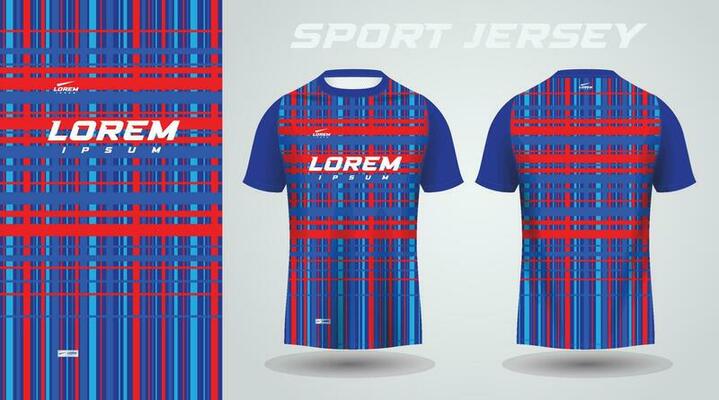This color photograph features an advertisement for a sports jersey from the placeholder text company "Lorem Ipsum." The image is divided into two sections: the left third showcases a check pattern of intersecting light blue, dark blue, and red lines, with white text stating "Lorem Ipsum" prominently displayed. The right two-thirds of the image highlights both the front and back views of the jersey, which echo the left section's color palette with woven blue and red stripes. The jersey features royal blue short sleeves and a matching ribbed round collar. On top of the image, "Sports Jersey" is written in white text. The background is a light grey, accentuating the jersey and including a dark gradient shadow below it. The design details, including the intricate check pattern and vibrant colors, make the jersey visually distinctive and appealing.